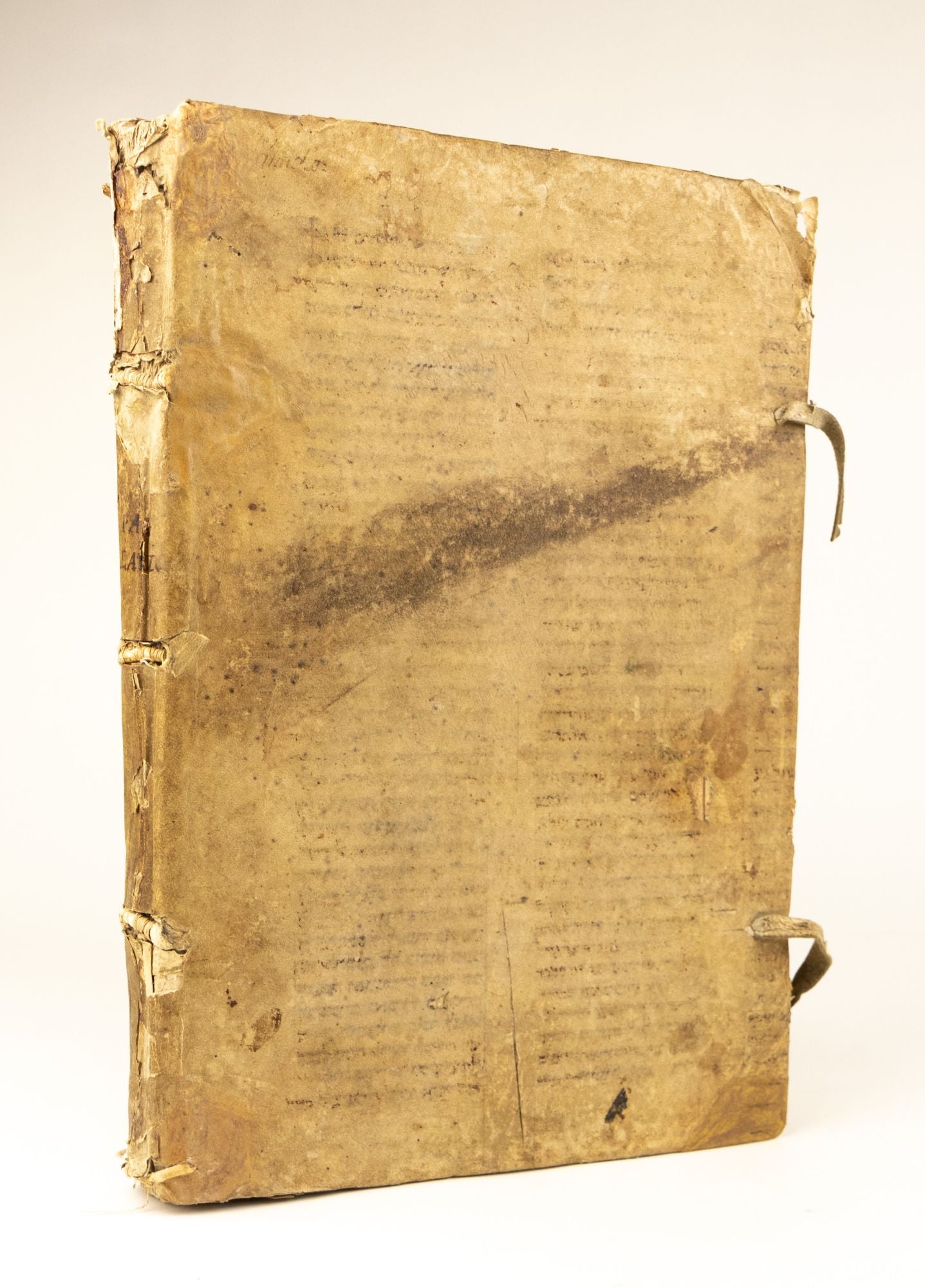This image features an ancient, well-worn book standing upright in front of a light pink and white background. The book is devoid of a cover and has visibly aged, with the pages having turned a deep brown over time, accented by some areas that have blackened. The binding on the left is barely holding together, with visible tears at the top and the right corner, exposing the fragile and torn pages underneath. The front page showcases blurred, illegible text, suggesting it once had printed material. Additionally, the book's surface exhibits a brown streak extending from the upper right, and a torn piece of paper protrudes from the bottom corner. A leather strap can be spotted at the top and bottom of the book, along with dark, indecipherable writing on the spine. The overall condition of the book indicates its ancient origins and extensive wear, with the top left corner of the spine ripped and the upper right corner of the cover bent, contributing to its crumbling, fragile appearance.